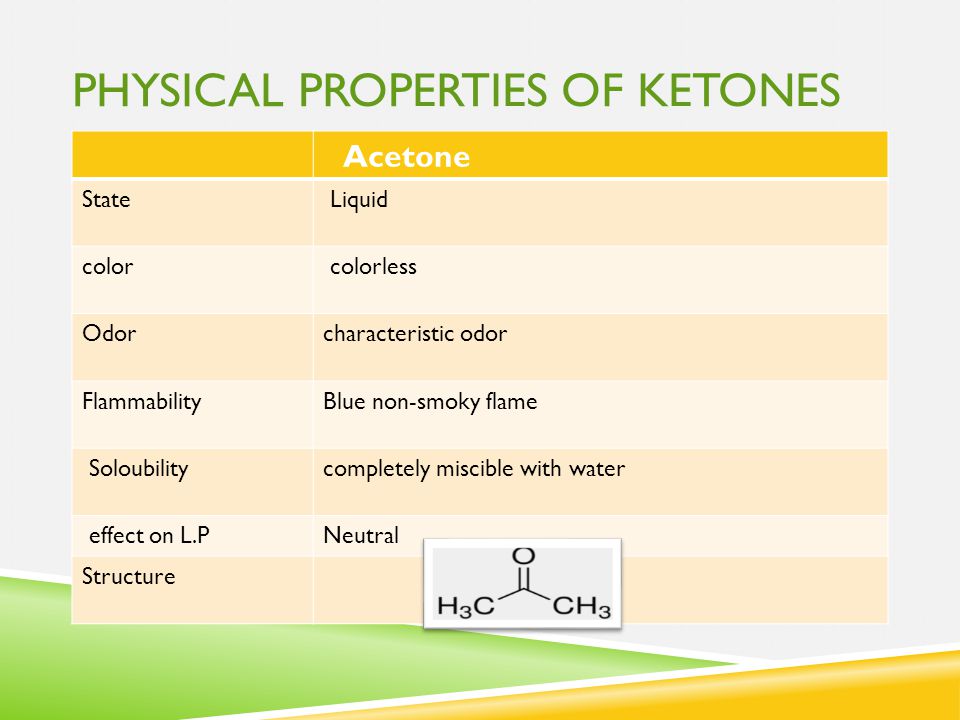The infographic titled "Physical Properties of Ketones" is displayed in green, all-cap letters against a gray background. The chart is organized in a table with black text, highlighting acetone in orange. Under the heading, it details various properties: 

- **State:** Liquid
- **Color:** Colorless
- **Odor:** Characteristic odor
- **Flammability:** Blue non-smoky flame
- **Solubility:** Completely miscible with water
- **Effect on LP:** Neutral

The chart includes the molecular structure of acetone with the chemical formula H3C-CO-CH3 and visual representation resembling a small, stick-figure-like diagram. The bottom portion of the table shows additional properties highlighted in green and orange, with a smooth, solid texture.